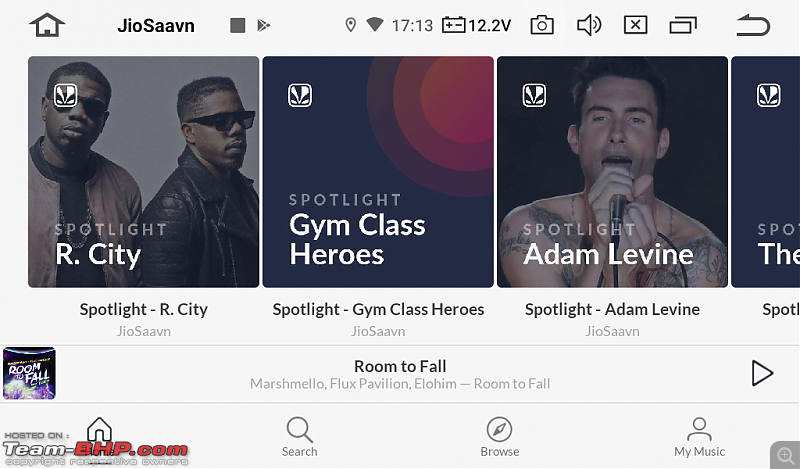This detailed caption describes a screenshot of a page from a mobile application:

---

The top left corner of the mobile application screenshot features a dark gray house icon. Next to it, in black text, appears the app name "GeoSavin" with specific capitalization: "G", "eo", "S", "av", "in". To the right of this text, there is a medium gray square, followed by a medium gray arrow logo with a white "X" through it. Further to the right, there are multiple icons, including, at the far right, a dark gray arrow icon that loops upward from the bottom and points to the left.

Below these icons, three tiles are displayed horizontally. Each tile has a white icon at the top left, featuring a square outline with rounded corners and a psychedelic abstract illustration in the center. From left to right, these tiles are labeled in large white text at the bottom left, with light gray text above each label: 
1. "Spotlight, Our City"
2. "Gym Class Heroes"
3. "Adam Levine"

Underneath each tile, additional information is provided in black text followed by light gray text: 
1. "Spotlight, Our City, GeoSavin"
2. "Spotlight, Gym Class Heroes, GeoSavin"
3. "Spotlight, Adam Levine, GeoSavin"

Below the tiles, a row of information is displayed. On the left, an album cover features dripping pink or purple text that reads "Room to Fail." In the center, the album title "Room to Fall" is displayed in black text, with the artists "Marshmallow, Flux Pavilion, Elohim" listed below in light gray text, followed by the song title "Room to Fall." On the far right of this row, a dark gray arrow points to the right.

---
This caption provides a comprehensive and detailed description of the elements present in the mobile application's screenshot.